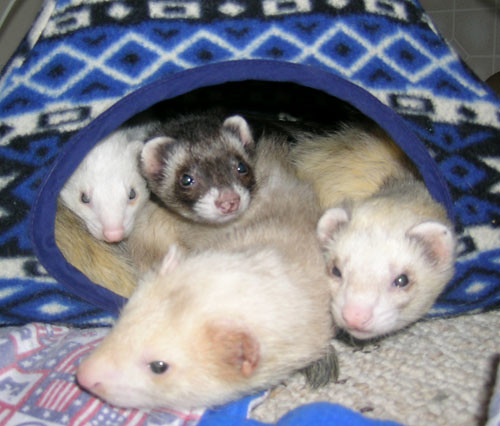The image depicts a cozy gathering of four ferrets nestled inside a fabric blanket or sweater, which features a detailed pattern of blue, black, and white designs, including rectangles, stripes, squares, diamonds, and chevrons. The oval opening of the cloth reveals the ferrets huddled close together, exhibiting a mix of colors: one ferret is white, another has a black and brown face, and the remaining two are a blend of brown, gray, and white. The ferrets' eyes shine in the camera flash, emphasizing their closed mouths and half-circle ears that add to their soft, endearing appearance. The entire scene rests on what appears to be a sheet resembling an American flag pattern, contributing to the snug and intimate setting.